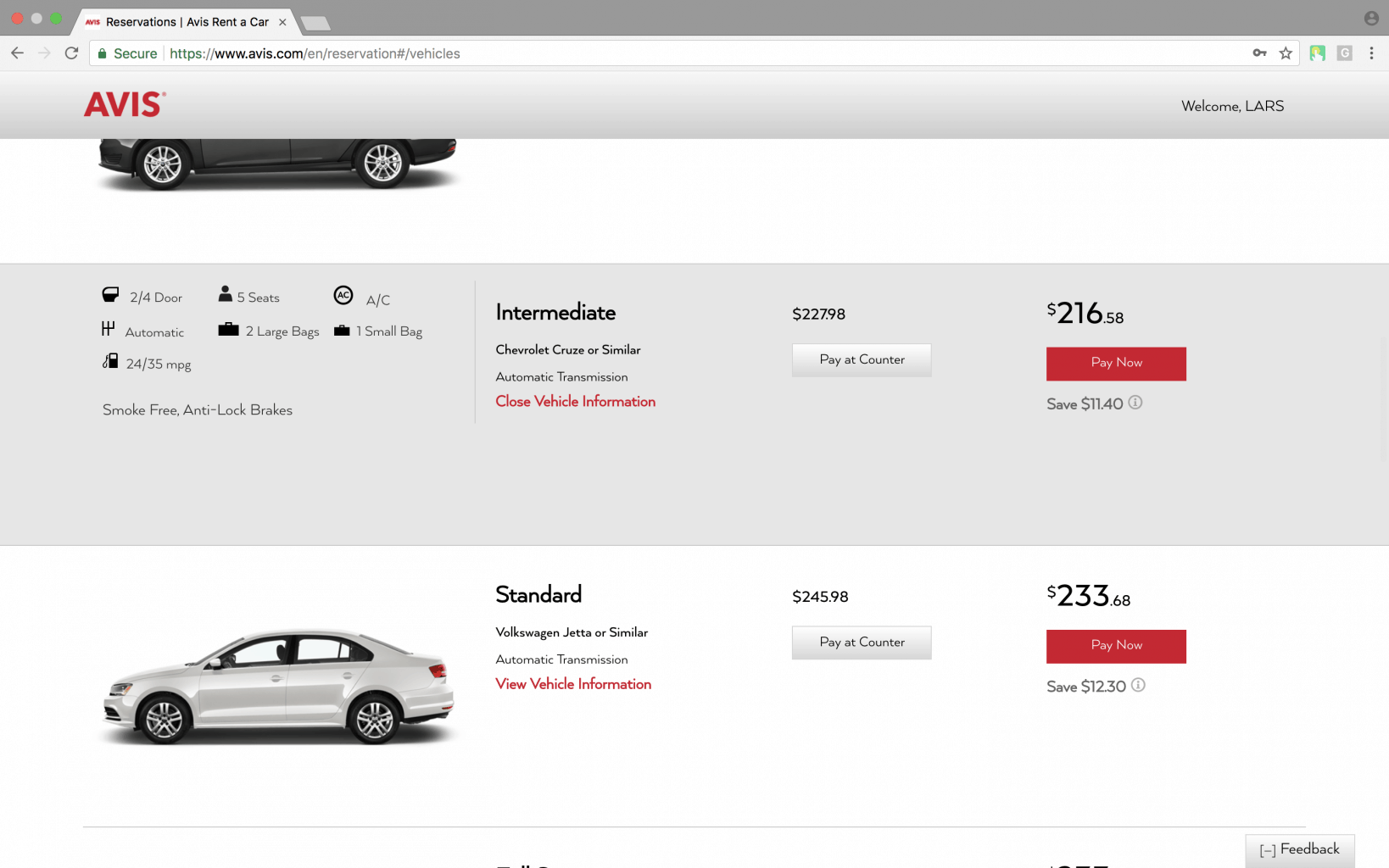The image showcases the Avis car rental website with a clean, user-friendly interface. The background colors are a mix of light gray and white. At the top, there's a navigation bar featuring a search tab for locating Avis cars and the site's URL, prominently displaying the "Avis" logo in bold, red capital letters (A-V-I-S). To the right of this bar is a personalized greeting, "Welcome Lars."

Below this section, there's a partial image of a black Chevrolet Cruze sedan. Only the left side of the car is visible, including the wheels, a portion of the headlight, the lower part of the hood, and the trunk. A light gray box underneath the image provides details about the vehicle: it’s classified as a sedan, equipped with air conditioning, two airbags, and information on its highway mileage. It falls under the intermediate class category, available for rent at $216 per day.

Additionally, the website features another car option below the black sedan – a pearl white Volkswagen sedan. This standard class vehicle is priced at $245 per day. There is a "Pay Now" option available for both cars that allows customers to save money by paying upfront. Finally, a feedback button is located in the bottom right corner, inviting users to share their experiences with the site.